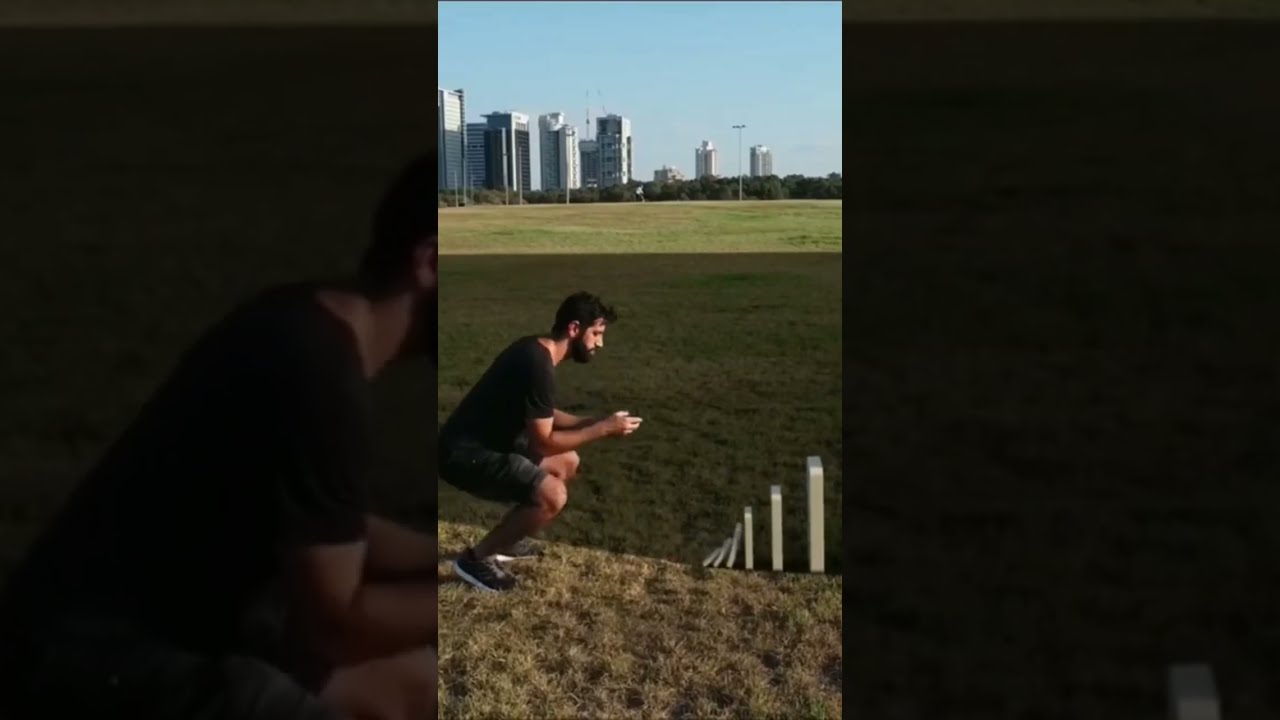In a large, green grassy field within a metropolitan area, a man of likely Asian descent is crouched on his toes, facing the right side of the camera. He is engaged in a dynamic activity, involving a series of large dominoes that vary in size, seemingly in the process of falling over. The man, sporting a beard, black hair, shorts, and a dark-colored t-shirt, appears to be initiating a dramatic domino effect. The background features the same image, zoomed in and faded on both the right and left sides, giving prominence to the main inset picture. Far in the distance, roughly half a kilometer away, city skyscrapers punctuate the horizon under a blue sky, partly illuminated by sunlight, creating a picturesque scene likely captured in a park during the afternoon.